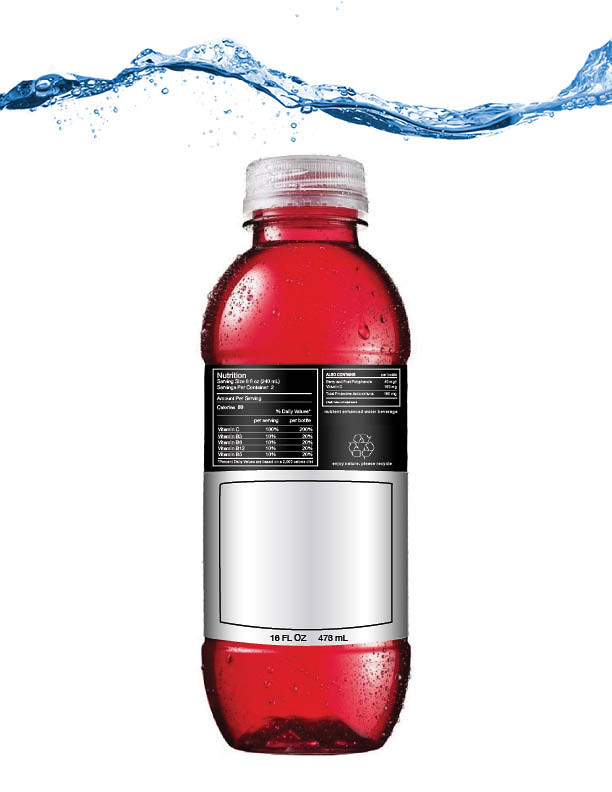This promotional image showcases a beverage against a clean, white background. At the top, a wave of blue water creates a dynamic motion, complete with small bubbles, adding a refreshing and lively feel. Positioned below the blue wave is a clear bottle filled with a vivid red liquid. The bottle features a clear screw-on cap, enhancing its sleek design. It also boasts a silver and black label; the silver portion has a black-bordered square with "16 fluid ounces" at the bottom, though it remains blank inside. The black section of the label includes a nutritional facts panel in white print, though the text is too fine to be legible.